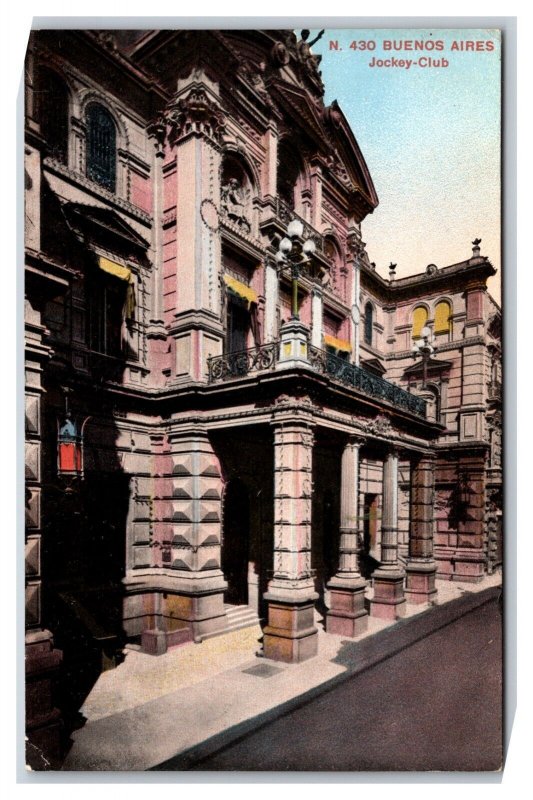This detailed photograph captures the exterior of an aging cement building, prominently labeled "430 Buenos Aires Jockey Club" at the top in red. The building's facade is a mix of tan and pink hues, giving it an old, slightly worn appearance. It's quite tall, possibly spanning four stories, and features a variety of architectural elements that contribute to its ornate design. Vertical pillars frame the entrance, which includes a foyer-like area supported by four beams. The exterior walls showcase a combination of horizontal stripes and three-dimensional block paneling. At the top, a deck is bordered by intricate metal railings, though the roof itself is not visible due to the vertical nature of the photograph. A clear blue sky stretches above the building, contrasting with the grainy texture noted in the photo. In front of the building, a street and sidewalk are visible, anchoring the scene in an urban setting. The overall composition suggests a historic and significant structure, possibly related to the Buenos Aires Jockey Club, with a visually compelling facade marked by stark contrasts and detailed ornamentation.